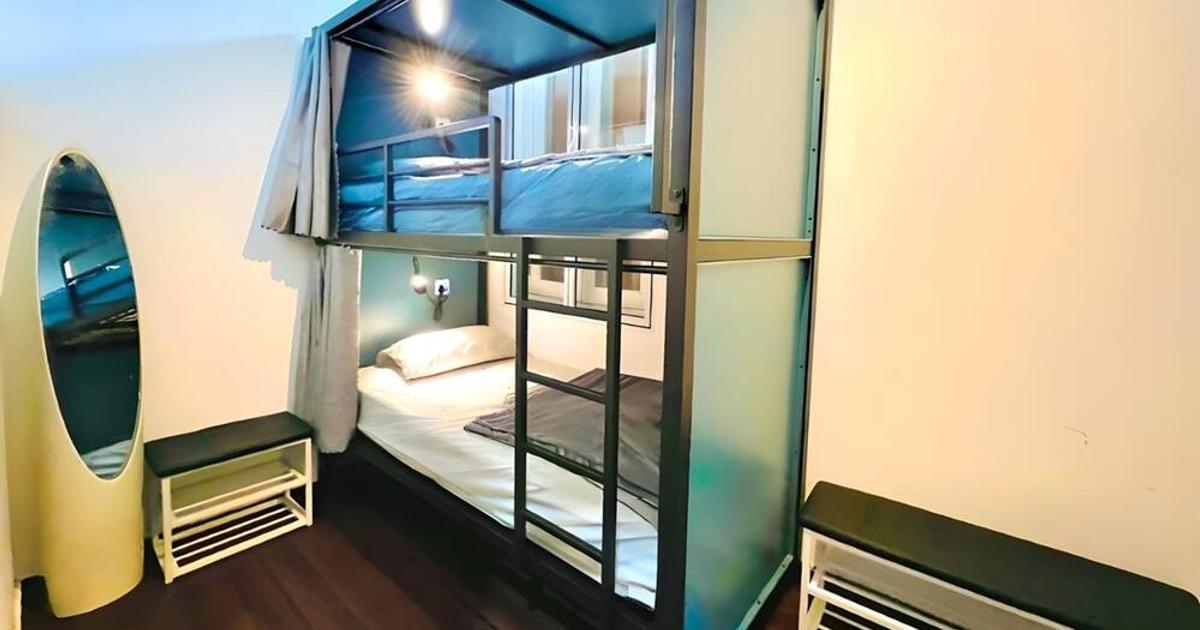This image depicts a small, sparsely furnished backpacker-style hotel room with two metal-framed bunk beds positioned under a window. The room's walls and ceiling are uniformly white, contributing to its bare, minimalist feel. The bottom bunk features a white mattress with a folded black sheet at the foot, complemented by a white pillow and an attached hanging light for reading. The top bunk has a blue mattress and is also equipped with its own light and a safety railing. Both bunks are outfitted with heavy blue canvas curtains for privacy.

A black metal ladder provides access to the top bunk, and an oval standing mirror is placed in the bottom left corner of the room, reflecting the lower portion of the bottom bunk. Adjacent to the mirror is a small stool with a white slatted design, doubling as a shoe rack. To the right of the bunk beds, another, longer black-top stool with white sides serves a similar function, adding to the room's practical yet austere décor.